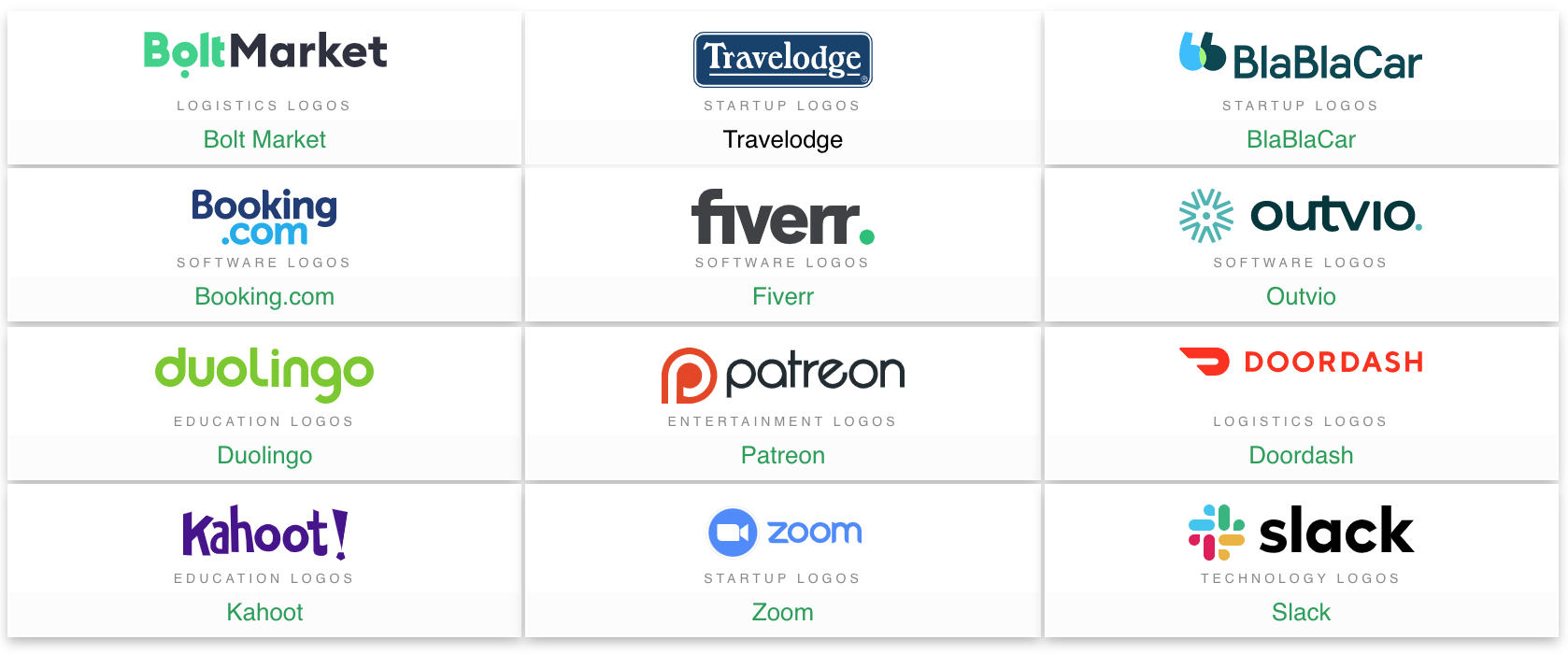The image depicts a screenshot featuring a grid of selectable websites organized in a three-by-four format. Each cell of the grid is labeled with a website name and its corresponding category of logos, meticulously arranged from left to right and top to bottom. 

**First Row:**
1. **Bolt Market** - Linguistics Logos for Bolt Market.
2. **Travelodge** - Startup Logos for Travelodge.
3. **BlaBlaCar** - Startup Logos for BlaBlaCar.

**Second Row:**
1. **Booking.com** - Software Logos for Booking.com.
2. **Fiverr (5RR)** - Software Logos for Fiverr.
3. **Outvio** - Software Logos for Outvio.

**Third Row:**
1. **Duolingo** - Educational Logos for Duolingo.
2. **Patreon** - Entertainment Logos for Patreon.
3. **DoorDash** - Logistic Logos for DoorDash.

**Fourth Row:**
1. **Kahoot** - Educational Logos for Kahoot.
2. **Zoom** - Startup Logos for Zoom.
3. **Slack** - Technology Logos for Slack.

Each cell succinctly indicates the website name followed by the type of logos attributed to that website, providing a clear and organized overview of the available options.